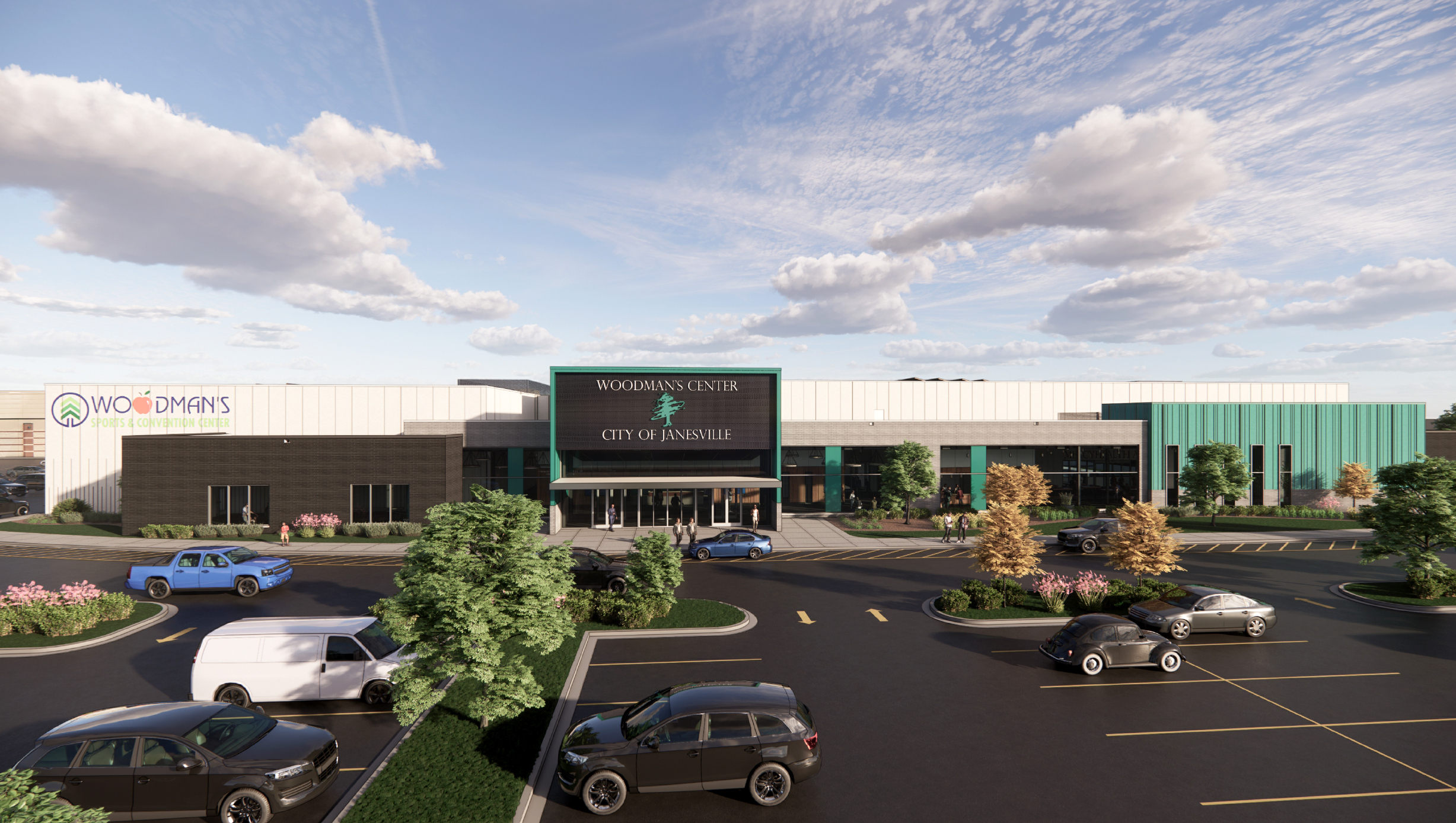The photograph, taken during the day and possibly from a drone, captures an expansive view of a new parking lot with a few cars, including a notable black Volkswagen Bug, a white van, a blue pickup truck, and some dark sedans. The freshly paved parking lot surrounds a large, long, warehouse-like building, with varied sections in green, white, and brown. The building bears the signage "Woodman's" with the second 'O' depicted as an apple, indicative of its function as a grocery store. Additionally, there's signage reading "Woodman's Center City of Janesville" accompanied by a tree logo. The scene is complemented by landscaping elements such as trees, grasses, and flowering plants, enhancing the parking lot's appearance. The background features a bright blue sky adorned with streaky white clouds.